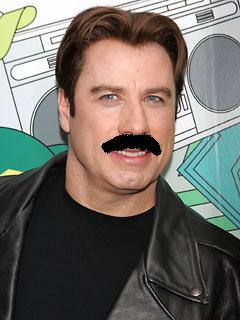This image features a small, highly stylized photograph of John Travolta. He appears from the head and shoulders to the top of his chest, with a short haircut and dark brown hair parted in the middle. Travolta is smiling or possibly in mid-speech, directing his gaze slightly away from the camera. Notably, he sports an unnaturally black mustache that looks digitally added, possibly through a simple software like Microsoft Paint, giving it an exaggeratedly phony appearance. He is dressed in a black t-shirt layered under a black leather jacket, complete with black buttons. Behind him, the background showcases a cartoonish boombox in shades of white and gray, featuring darker gray speaker ports. This is set against a backdrop decorated with various teal-green lines and shapes, adding an abstract and playful element to the image. Travolta's clear skin and minimal wrinkles suggest he is in his late 40s.